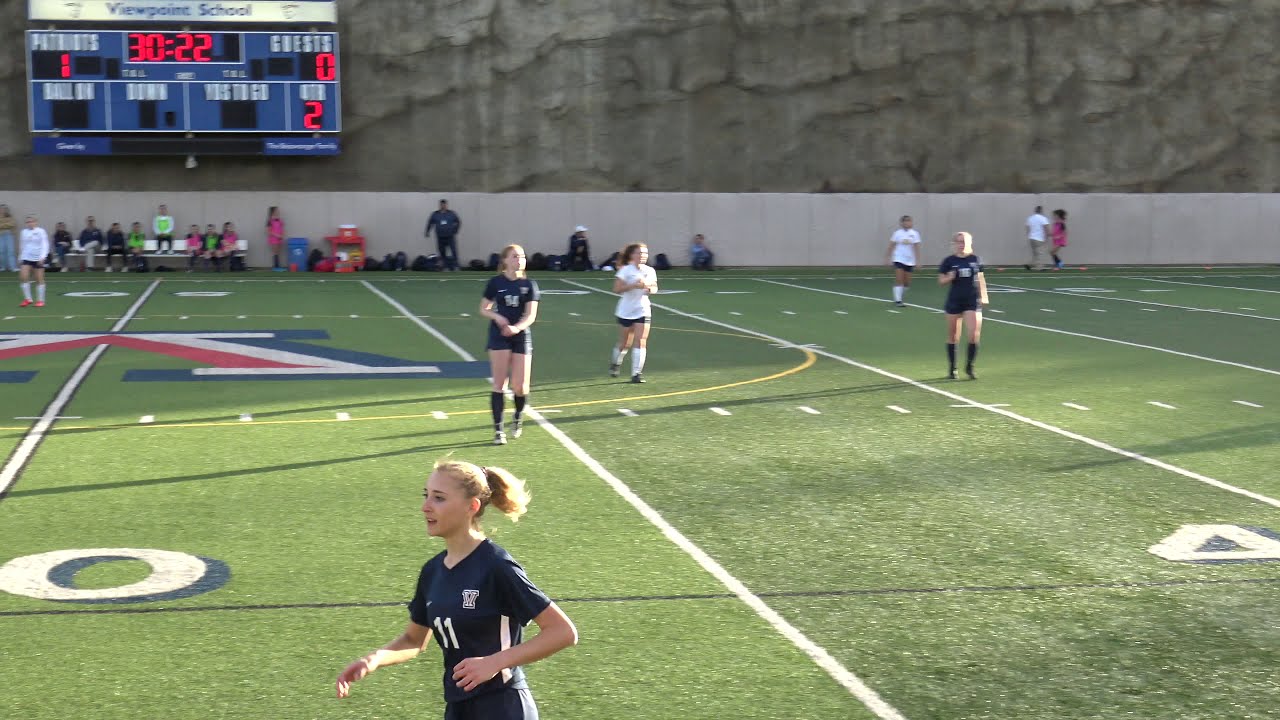This horizontally aligned rectangular image depicts a high school or college soccer match between two women’s teams, the Patriots and the Guests. The field features green artificial turf, striped with white lines and accented with red and blue markings at the center. In the foreground, a player from the Patriots, identifiable by her navy jersey and blonde ponytail, is running towards the left. Her team leads 1-0 as indicated by the scoreboard in the upper left corner, which reads "Viewpoint School" and shows a time of 30 minutes and 22 seconds in the second quarter. The background displays a large brown stone wall at the top, with a shorter light gray or white stone wall running horizontally across the picture. Spectators and coaches, dressed in casual t-shirts rather than uniforms, are seated along the white stone wall, observing the game.